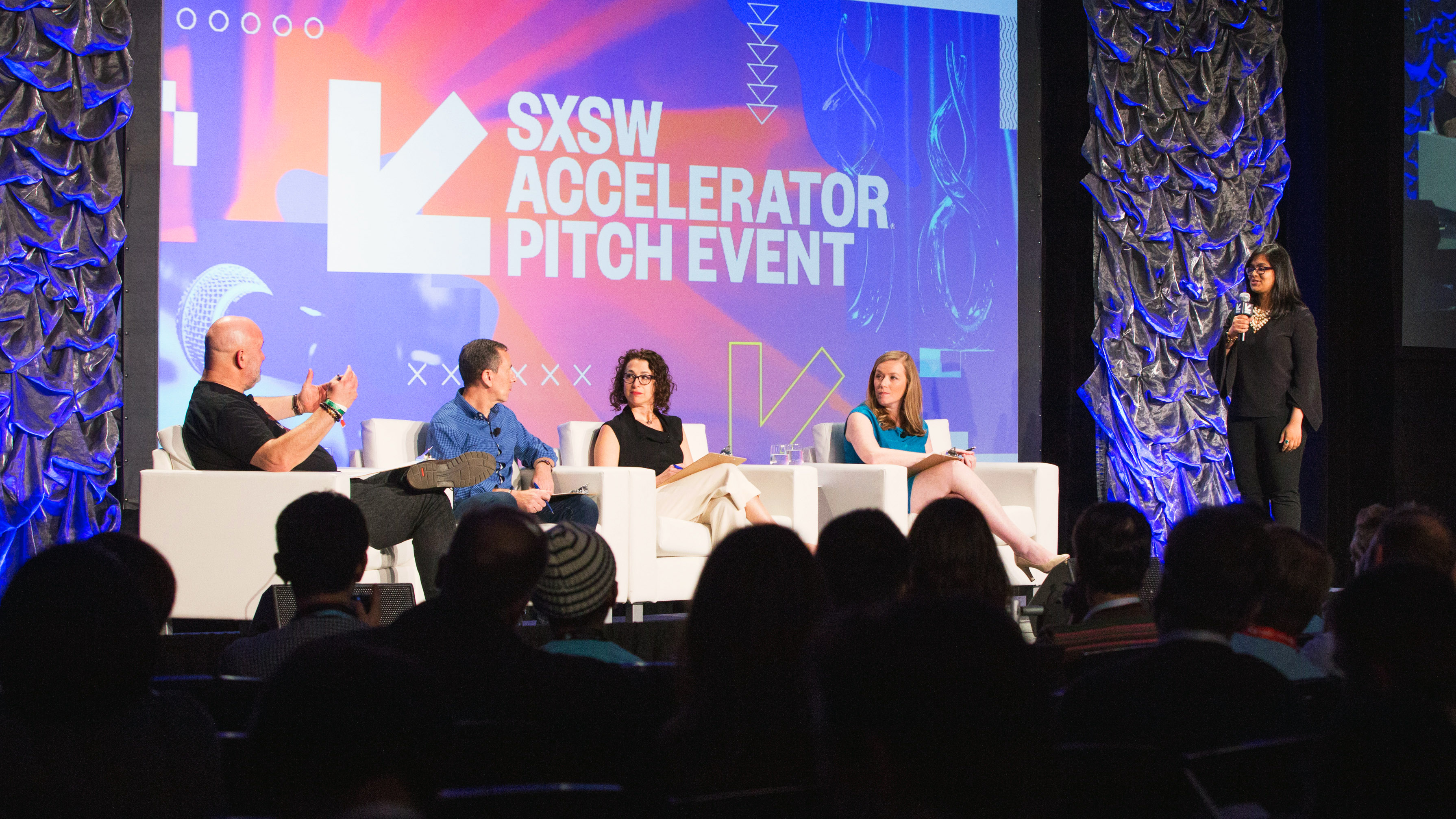This high-quality professional image captures a live moment from a South by Southwest (SXSW) Accelerator Pitch event held in a studio-like setting, dimly lit except for the brightly illuminated stage. The focal point of the stage is a large, colorful screen that prominently displays the text "SXSW Accelerator Pitch Event." Flanking the screen are elegant fabric decorations that drape the wall, adding a touch of sophistication to the ambiance.

On stage, four ivory chairs are arranged in a semi-circle, each occupied by a person engaged in an active discussion. The two men to the left and two women to the right are all professionally dressed, reflecting their diverse roles and backgrounds. An older, bald man wearing a black shirt and bracelets is speaking animatedly to the group. Next to him, a younger man in a button-up blue shirt and black pants listens attentively. 

The women seated to the right are also professional in their appearance—one in a black outfit and glasses, with blue and white pants, and the other wearing a teal dress with longer brown hair. Nearby, a woman dressed entirely in black stands to the far right of the stage, acting as a moderator. She holds a silver microphone and sports medium-length black hair, glasses, and a pearl necklace.

The viewpoint of the photo is from behind the audience, whose shadowy profiles are visible, creating a sense of anticipation and engagement. The dynamic setup and polished decor highlight the event's formal yet interactive atmosphere.